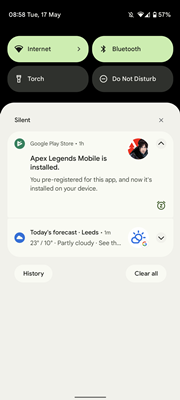This screenshot captures a smartphone's operating system interface. At the top, a slightly blurry bar displays essential phone data, including the date (Tuesday, 17th of May) and the time. Adjacent indicators show signal strength, battery level (57%), and WiFi signal strength. Below this, four toggle buttons are aligned in a row. The first two, labeled "Internet" and "Bluetooth," are light green with black text indicating they are active, while the next two buttons, "Torch" and "Do Not Disturb," are in gray, denoting inactive status.

Beneath these toggles, a gray background supports a white overlay containing search results. Featured prominently is a Google Play Store notification in dark letters indicating that "Apex Legends Mobile" is installed, accompanied by a small, colorful, but indiscernible icon. It also mentions that the user was pre-registered for this app.

Further down, a weather update for Leeds is provided, showing a current temperature of 23 degrees Celsius with a low of 10 degrees, partly cloudy conditions, and a small weather icon depicting the sun peeking behind clouds. Beneath this forecast are two small radio buttons, followed by two menu items: "History" on the left and "Clear All" on the right.

The bottom portion of the screenshot is mostly vacant, consisting of a large gray area that takes up about one-third of the image.